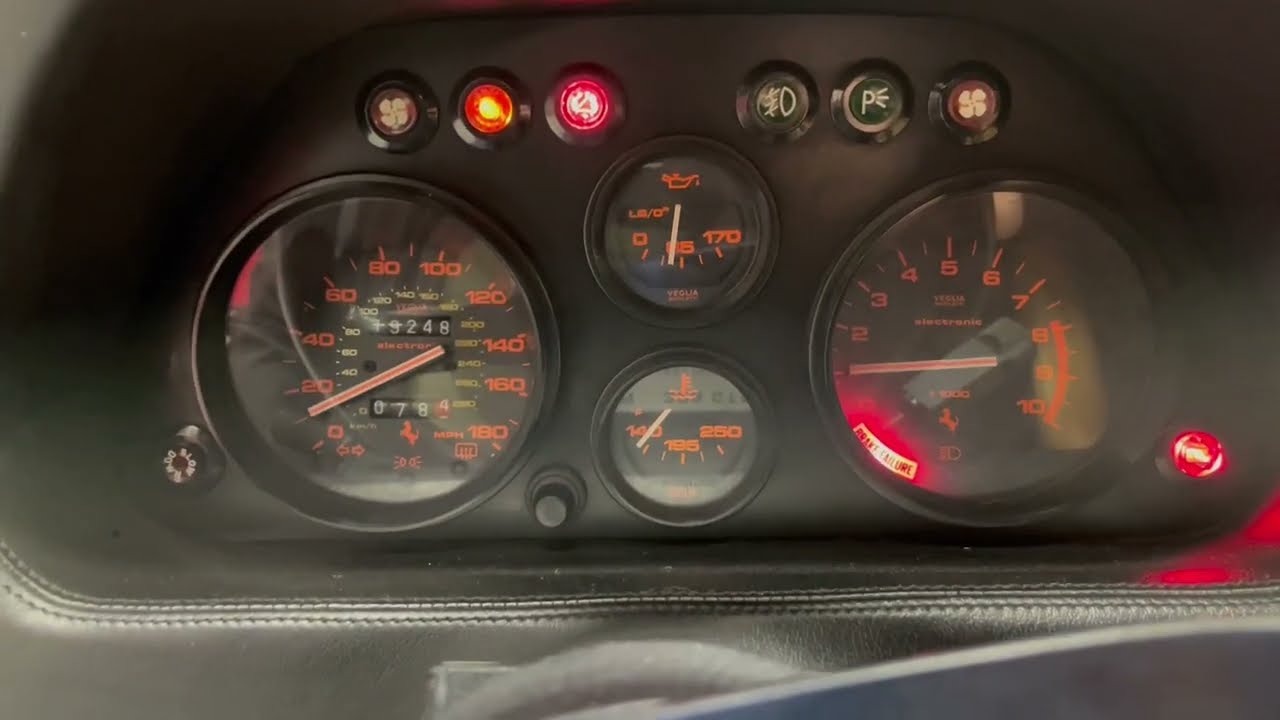The image depicts the interior of a car, focusing on the black leather dashboard with a distinct retro look. Prominently featured from left to right are several gauges: an analog speedometer with red numbers ranging from 0 to 180 and a red indicator pointing at 10 miles per hour; two smaller dials in the center—one for oil temperature marked from 0 to 170, and the other for another temperature-related function displaying numbers from 140 to 280; and a larger gauge likely representing the odometer or tachometer. Positioned above the gauges are six indicator lights: one resembling a fan, another glowing red, a third also glowing with a fan-like symbol, followed by three more buttons with various symbols, including one that represents the letter 'P' and another for a headlight. The overall design combines practicality with a classic aesthetic, underscoring both form and function.